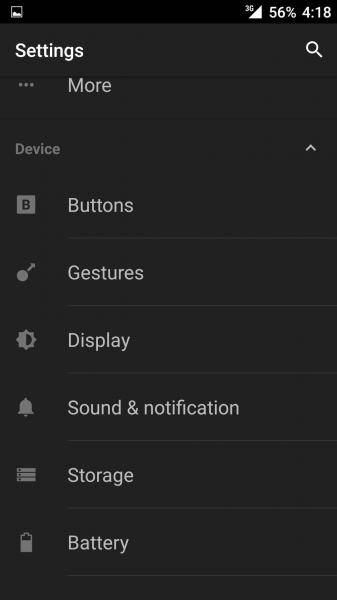A detailed screenshot of a phone's settings menu is depicted against a black background. In the top right corner, symbols indicate the phone’s status: a “3G” network, a battery at 56% capacity, and the number “418.” Below, a black banner features the word “Settings” in white, accompanied by a magnifying glass icon on the right.

Directly beneath, another white label reads “More,” with “Device” following below. The menu lists six options, each in white text and separated by thin white lines. The options are:

1. **Buttons**: Denoted by a “B” icon.
2. **Gestures**: Symbolized by a circle with an arrow pointing outward.
3. **Display**: Represented by a settings gear icon.
4. **Sound and Notification**: Marked by an alarm bell icon.
5. **Storage**: Indicated by a menu grid icon.
6. **Battery**: Shown with a battery icon partially depleted at the top.

No other content is present on this page.